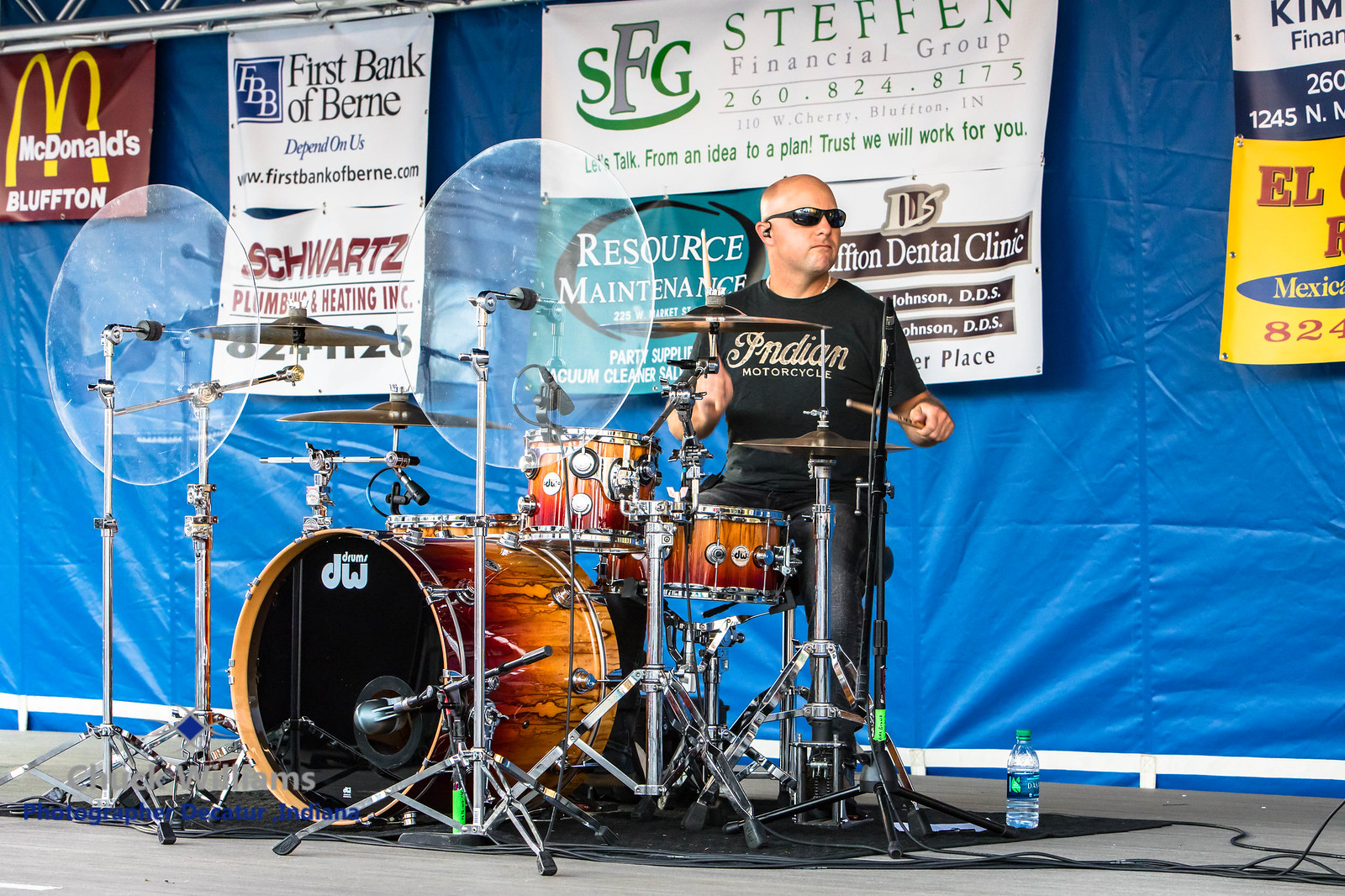The image captures a drummer, who is slightly balding and wearing black sunglasses, deeply immersed in his performance on a stage. He dons a black t-shirt emblazoned with "Indian Motorcycle" in gold letters. His drum set, showcasing a DW brand logo on the bass drum, features a rich orange color that transitions to a darker red hue. The kit is equipped with multiple snares, hi-hats, cymbals, and other drum accessories. There is a clear Dasani water bottle positioned near his feet, along with various cords scattered across the gray stage floor. Behind the drummer, a blue tarp-like backdrop is adorned with multiple sponsor banners including McDonald's, First Bank of Bern, Schwartz Plumbing and Heating, Steffen Financial Group, and Resource Maintenance, among others. These banners are mounted on a series of steel bars, adding to the local event ambiance where the drummer is performing.